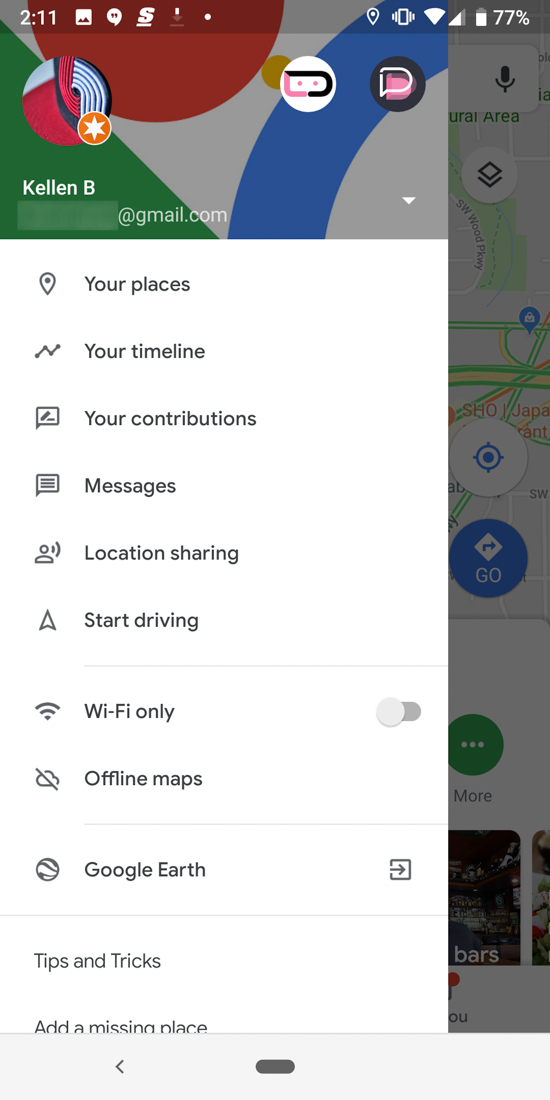The image showcases the main menu of a navigation application on an Android smartphone, predominantly occupying the left side of the screen. At the top left corner, the menu header displays "KLP" with the associated email address partially obscured by HTML elements. The menu background comprises a multi-color palette including green, blue, red, yellow, and white.

On the right side of the screen, several features are visible concurrently. Positioned at the top right is a map denoting the current location with a blue "Go" button nearby. Below the map, towards the bottom right, there are thumbnails of various places.

The site menu on the left contains several options, each listed sequentially:

- Your Places
- Your Timeline
- Your Contributions
- Messages
- Location Sharing
- Start Driving

Further down the menu is a toggle switch labeled "Wi-Fi only," which is currently off and displayed in grey. Additional menu items include "Offline Maps" and "Quickly Apps," accompanied by a greyed-out arrow button.

At the bottom of the menu, there are sections for "Tips and Tricks" and "Add a Missing Place."

This detailed depiction represents an interactive and colorful interface of a widely-used navigation application, quickly maps, on an Android device.